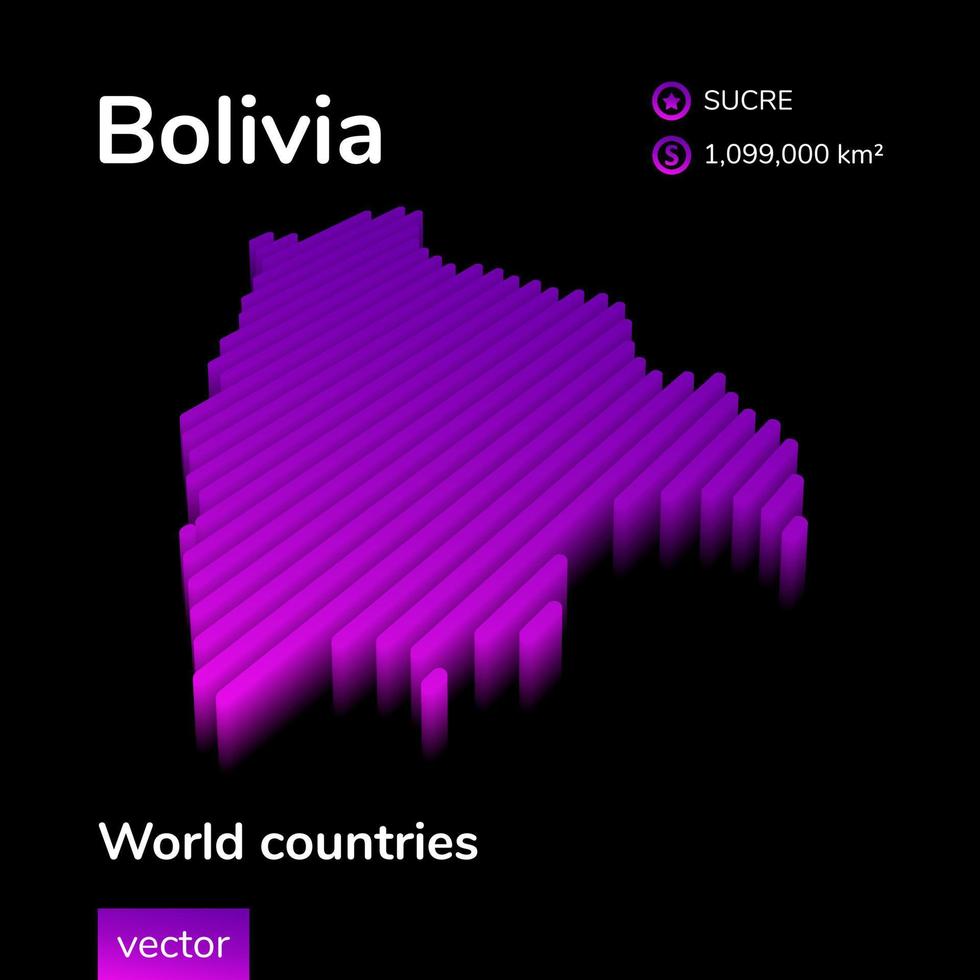The image is a highly stylized, three-dimensional digital representation of the country of Bolivia. The design features vertical, rectangular slices creating the map's form with slight black silhouette shading between each slice. A vibrant gradient transitions from a light purple at the bottom to a dark purple at the top. Positioned against a pure black background, the composition includes several distinct textual elements: in the upper left corner, the word "Bolivia" is prominently displayed in white text; to the upper right, "Sucre" appears beside a purple circle containing a star, with the country’s area, "1,099,000 km²," written below in white, accompanied by a purple circle with a dollar symbol. In the lower left corner, "World Countries" is inscribed in white text above a small rectangular purple box labeled "Vector."